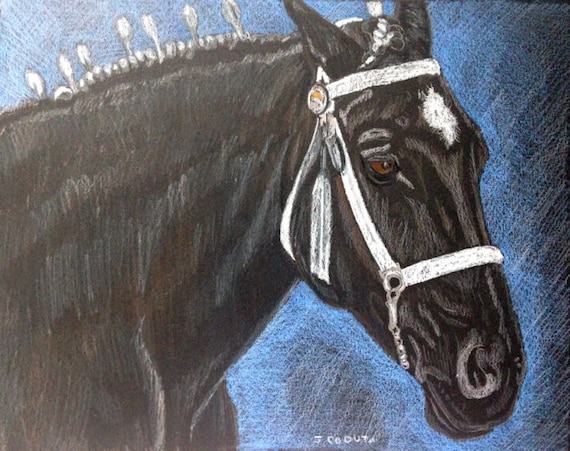This image is a drawing of a muscular black horse with a lighter brown and white patchwork. Prominently, he has a large white diamond marking on his forehead and light brown eyes that gaze pensively to the right. The horse's mane, which is white with hints of black and brown, appears well-groomed with some strands sticking up, as if prepared for a competition. He is wearing a white bridle that includes a harness around his nose and a chain around his ears, keeping his mouth closed. The background is a gradient of various shades of blue with darker patches, enhancing the depth and mood of the image. This artwork seems to be done in colored pencils, suggesting a blend of fine detail and soft texture. At the bottom of the image, the artist’s name, likely "Jay Cebuto" or a similar variation, is inscribed, though it's slightly unclear. The drawing looks like it could be the work of an older child or teenager.